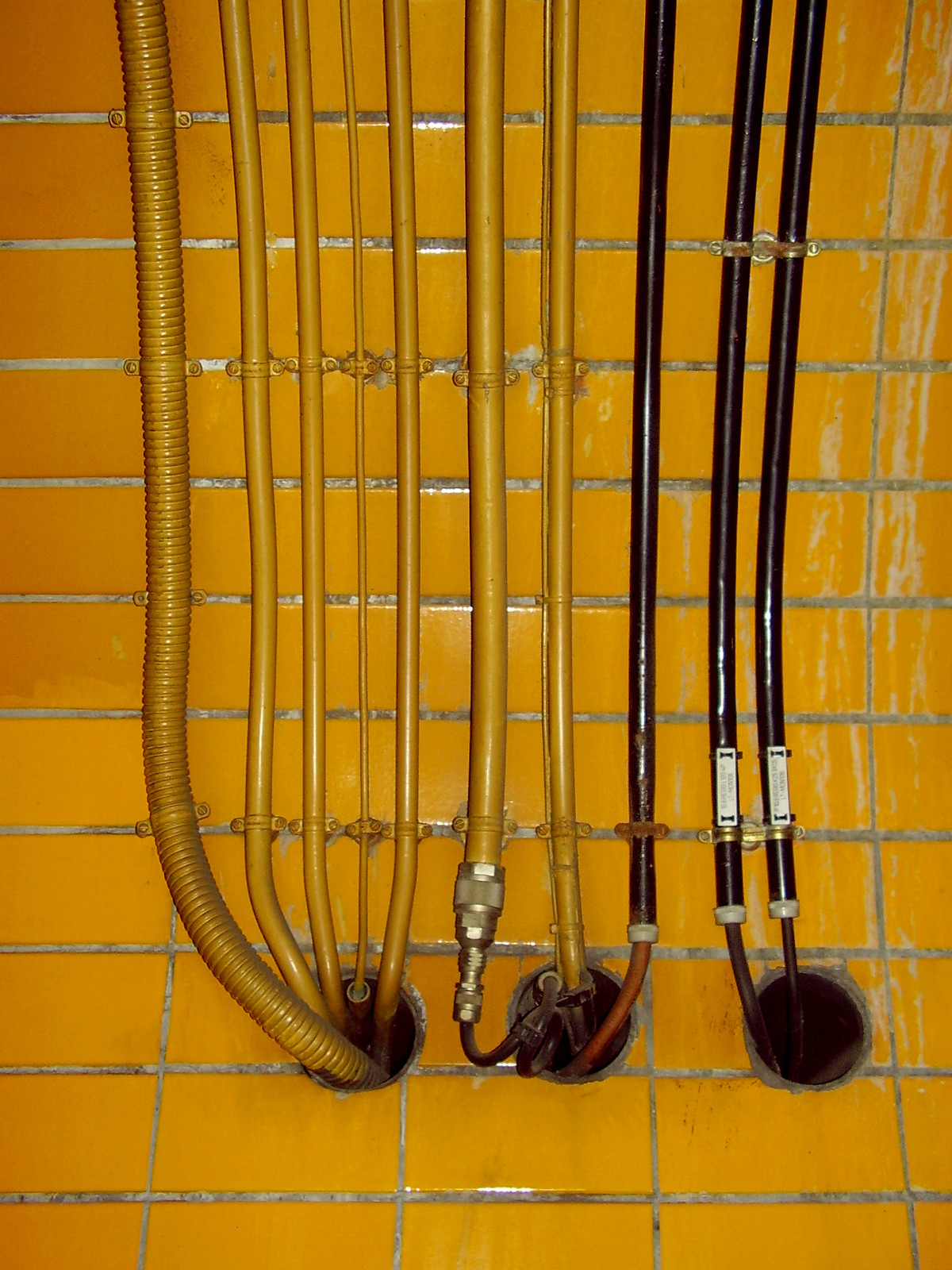This indoor colored photograph captures a vertically aligned rectangular scene, showcasing a yellow-orange tiled surface reminiscent of a gym bathroom or shower wall. The tiles are separated by grody, grayish caulking. The image features three large holes along the bottom edge of the scene, each with an array of pipes protruding and extending vertically upwards to the top of the picture. In the first hole, there are two black pipes. The second hole contains three pipes, with one black pipe and the other two closely matching the tile's color. The third hole is densely packed with five pipes of varying sizes, with the one second to the left being notably thin, while the far-left pipe is thick, gold-colored, and appears corrugated or ribbed. The remaining pipes exhibit smooth exteriors, with approximately six showing gold hues and three black ones positioned towards the right, connecting to brown tips near the holes. Each pipe’s placement and material hint at a maze of functional piping disappearing into the ambiguous space between a floor or a wall.